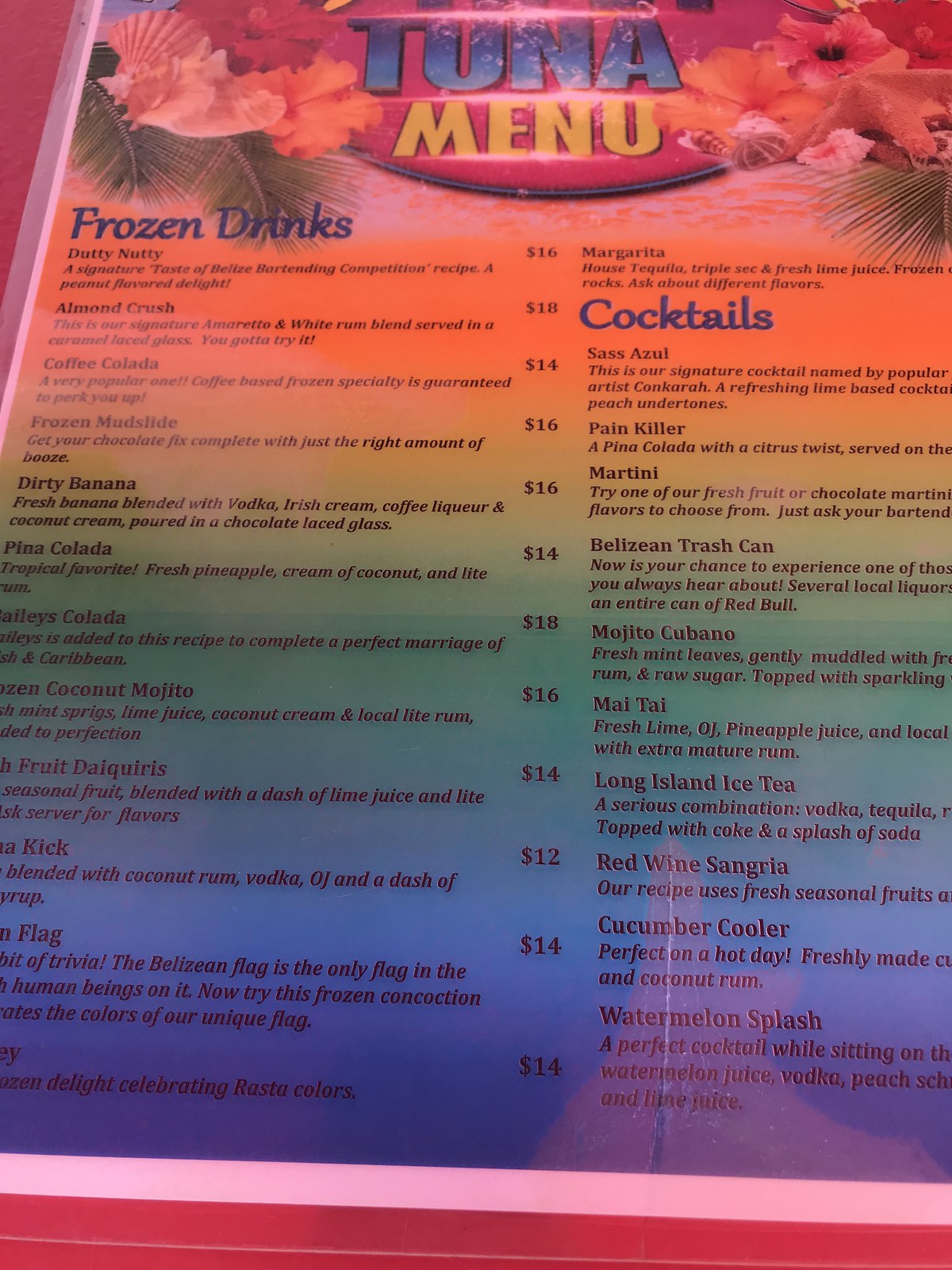The image is of a vibrant, laminated menu titled "Tuna Menu," which features two sections: frozen drinks on the left and cocktails on the right. The menu showcases a gradient, rainbow-themed background transitioning from orange at the top to yellow, green, blue, and ending with purple at the bottom. The lamination gives the menu a glossy finish, adding a touch of shine. Decorative floral illustrations adorn the top of the menu, enhancing its aesthetic appeal. The frozen drinks are priced between $12 and $18. The cocktail section lists various options, including Sass Azul, Painkiller, Martini, Belizean Trash Can, Mojito Cubano, Mai Tai, Long Island Iced Tea, Red Wine Sangria, Cucumber Cooler, and Watermelon Splash, though the prices are not visible in the image.